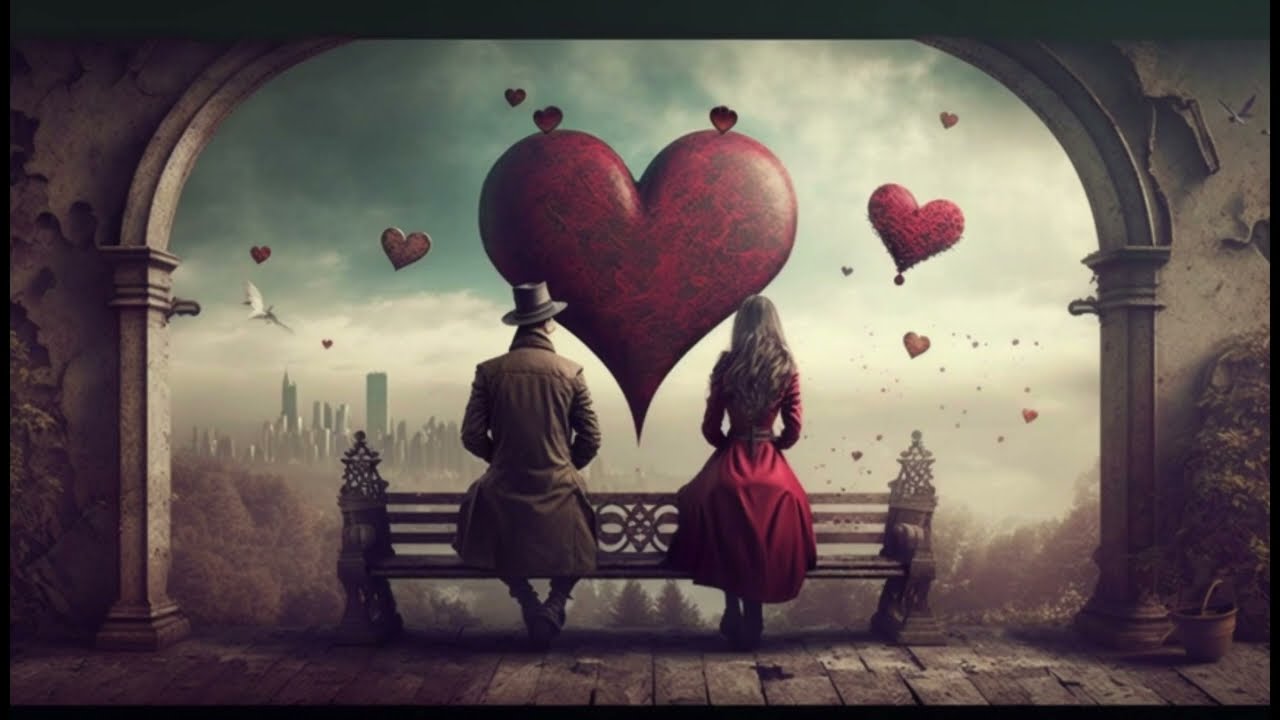In this AI-generated, surrealist, steampunk-themed image, a man and a woman are seated on an old-fashioned wrought iron park bench within a dilapidated, early 1900s-style building. The interior features crumbling walls with peeling and cracked paint, and a rough, broken stone-tiled floor. The bench appears to face the viewer, but the couple is seated as if their legs have been slid through the lower slat—a visual trick that adds to the surrealism of the scene.

The man, dressed in a tan trench coat and a gray fedora, sits next to the woman, who wears a long, red dress with wavy brown hair cascading down to her waist. The archway they are sitting in front of opens to a murky, smoggy landscape with an obscured city skyline, filled with skyscrapers and buildings that peek through the haze. 

In front of the couple, a large, red and black marble-textured heart floats somberly, and smaller hearts drift through the sky, adding a dreamlike quality. To the left of the archway, an unhealthy-looking tree and some leaves are visible, contributing to the gloomy atmosphere. The overall scene evokes a sense of decay mixed with elements of love, underpinned by a steampunk aesthetic that makes the image intriguing to examine.